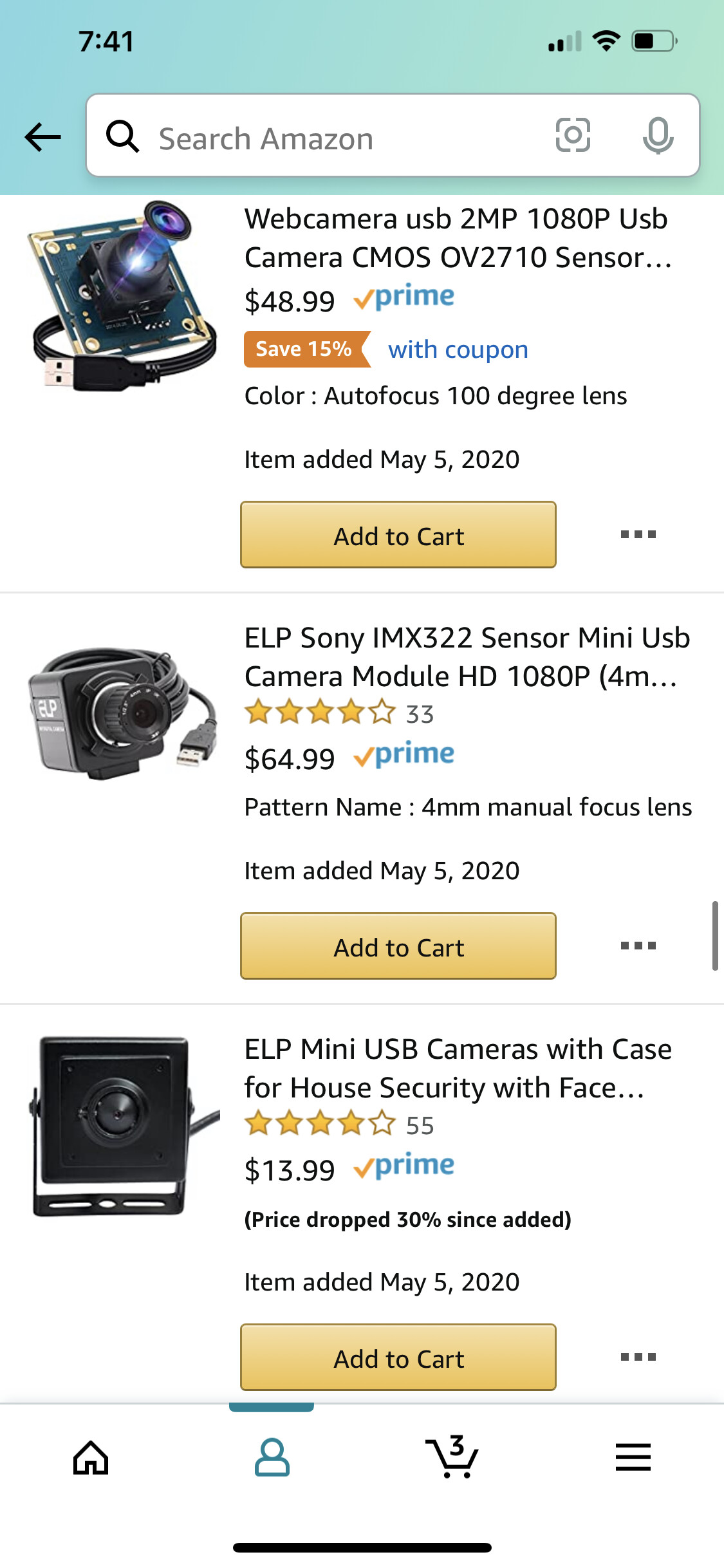A screenshot from a mobile device depicting a vertical list of webcam products available on Amazon. At the top of the screen, a search bar with the text "search Amazon" and a search icon is clearly visible. Below the search bar, three different webcams are displayed in a list format.

Each webcam entry consists of a product image on the left and a descriptive text on the right. The first product is a "USB 2 MP 1080p USB Camera," currently offering a 15% discount with a coupon. The second product listed is the "ELP Sony IMX 322." The third item is the "ELP Mini USB Camera with Case."

At the bottom of the screenshot, a navigation menu bar includes icons for home, profile, and a shopping cart. Notably, the shopping cart icon indicates that it contains three items.